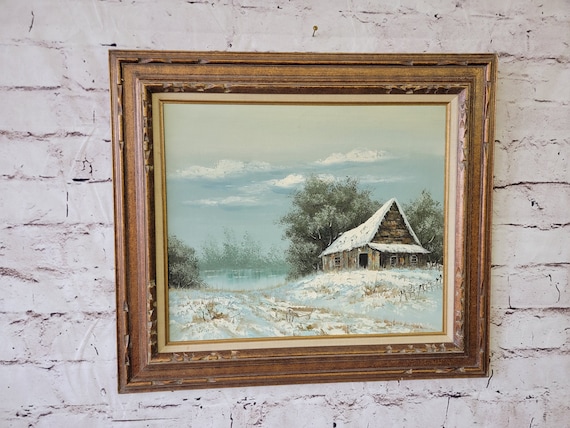The image captures an old, whitewashed brick wall, with visible gaps and wear, serving as the backdrop for a painting encased in a basic brown to bronzy frame, slightly off-center to the left. The painting, possibly an old photograph due to visible wear on the frame, depicts a serene, snowy landscape. Dominating the right side is an apparently abandoned farmhouse with a snow-covered roof, nestled among snow-laden trees and bushes. Extending in the foreground is an expanse of snow-covered grass, leading the viewer's eye to a glistening lake at the center of the scene. The background reveals a cloudy sky, along with further scattered trees and foliage, enhancing the painting's depth and tranquility.